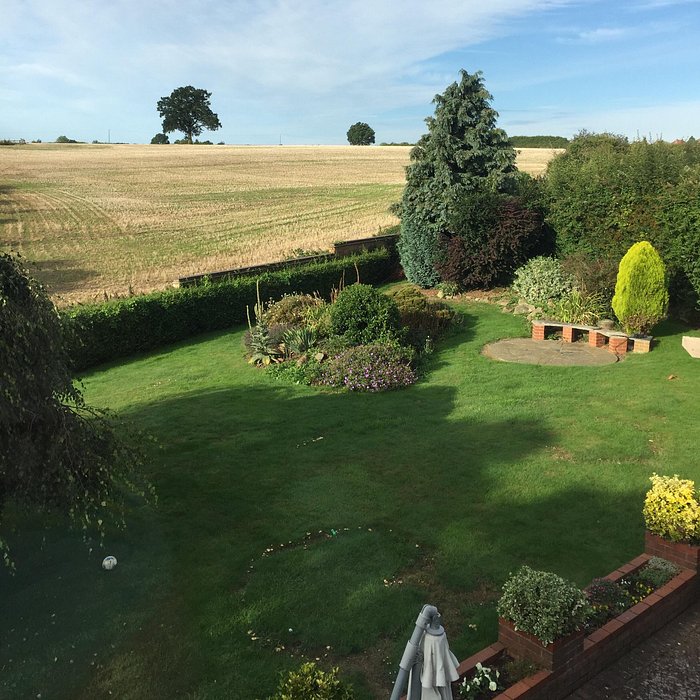This square-shaped, realistic photograph captures a picturesque countryside scene, possibly farmland, taken from a height of 20 to 30 feet at a slight angle. In the background along the horizon, there is open farmland with green fields and short beige-tan plants growing in neat rows. Scattered trees line the horizon under a bright blue sky with white, fluffy clouds.

In the foreground, a neatly landscaped backyard unfolds, featuring lush, green grass and various plants. On the right side, tall trees, including one resembling a Christmas tree, cast shadows on the lawn. Surrounding the yard, there are bushes acting as a natural fence, and additional small bushes of varying shades of green add to the greenery.

A brick planter with both green and yellow plants sits at the bottom right of the yard, alongside a bench presumably made from brick with rectangular boxes on top. A white platform, possibly part of a larger patio area, is also visible, creating a seamless blend of natural and constructed elements in this tranquil outdoor space.

Overall, the photograph showcases a harmonious blend of well-kept backyard elements with the expansive beauty of the countryside beyond, emphasizing the vivid greenery and calm atmosphere of the rural setting.